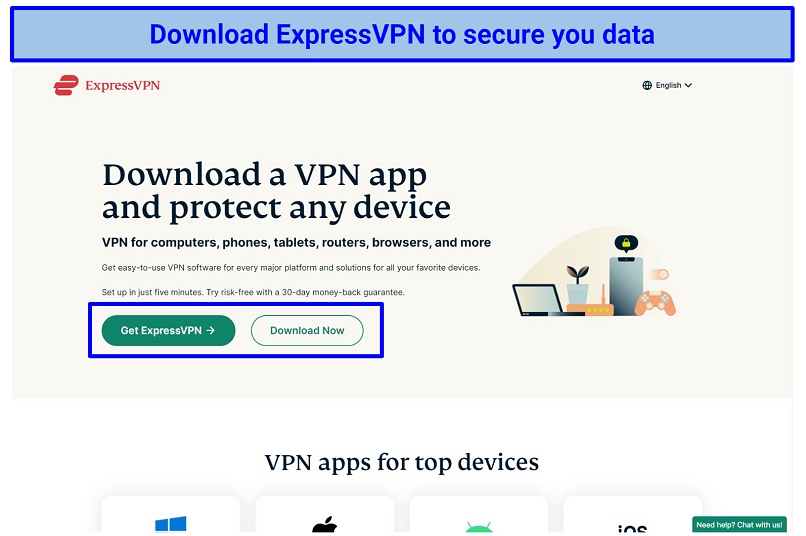The webpage for ExpressVPN features a prominent banner at the top in a neatly outlined blue square with a lighter gray interior. The banner employs a blue font that reads, "Download ExpressVPN to secure your data," accompanied by the ExpressVPN name in red and its logo on the left-hand side. 

To the right of this banner, there's a graphic element consisting of a gray circle representing the globe with intersecting lines, and just below it, a black arrow pointing downwards beside the word "English." Directly beneath this, black text on the left states, "Download a VPN app and protect any device," followed by a rundown of compatible devices: computers, phones, tablets, routers, browsers, and more.

In a more delicate gray font, additional details highlight the ease of use and wide-ranging compatibility of the VPN software, emphasizing its setup capability within five minutes and promoting a 30-day money-back guarantee. 

Below this informational section is a horizontal tricolor box in gray, red, and blue. This box includes a gray circle with white text that reads "Get ExpressVPN," marked by a white arrow pointing to the right, and a green circle with an internal white section and green text, asserting "Download now."

On the right side, there's an image of a laptop featuring an orange base, possibly with a computer interface on the screen. The image is accompanied by an illustration of Wi-Fi signals in orange and a game controller to the right.
 
Following this section, a white background houses a black-font heading that reads, "VPN apps for top devices." Beneath this heading, there are four partially visible boxes: the first displaying two blue squares, the second likely showing the Apple logo in black, the third featuring a light green half-circle with antenna-like extensions, and the fourth associated with iOS, marked by black text.

To the right margin, a green box with white font offers immediate assistance, stating, "Need help? Chat with us."